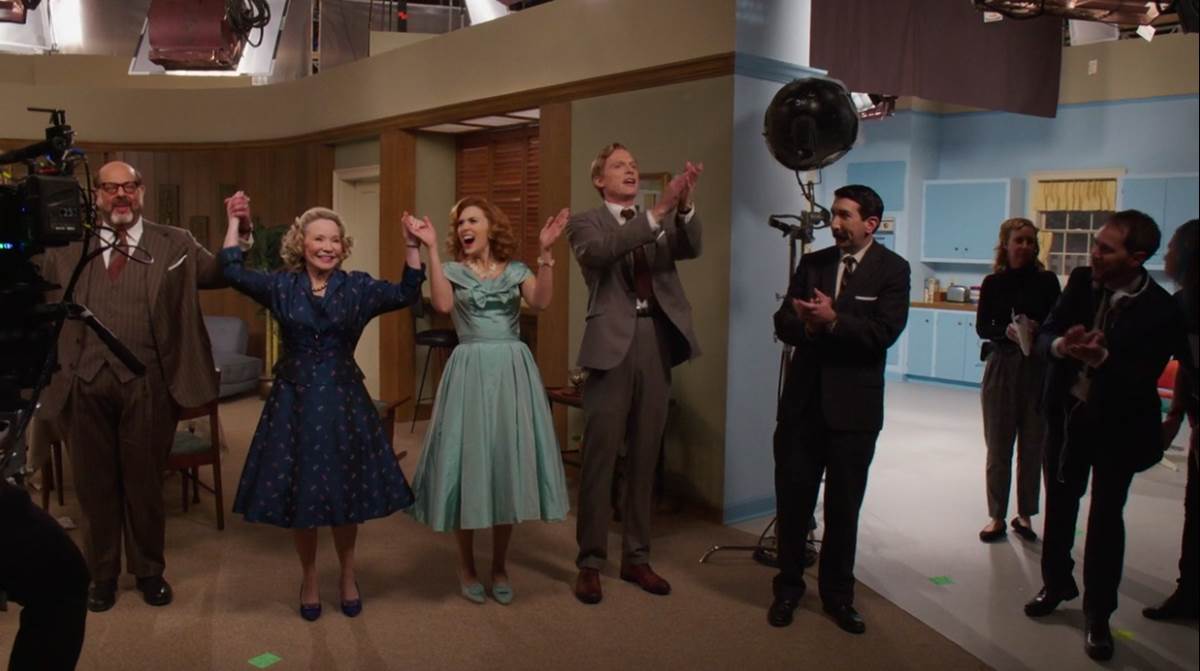This photograph appears to be a behind-the-scenes shot from the set of the television show WandaVision, reminiscent of a 1950s TV series. The central focus is on a group of eight people, including Elizabeth Olsen, who plays Wanda, and other cast members in period-appropriate 50s attire. Olsen is seen in a navy blue dress adorned with white polka dots, while another woman stands next to her in a long green dress with a bow at the front. The men in the scene wear brown suits, white shirts, and ties. They are all facing the camera with smiles, clapping with raised hands, evoking a celebratory mood as if wrapping up a scene or episode.

The set features a living room ambiance to the left with classic 50s decor, leading to what appears to be a kitchen on the right. The kitchen has a white floor, a brown countertop, and distinctive turquoise cabinets, with a window shade drawn in brown. Above, stage lighting and other production equipment are visible, hinting at the studio environment.

Adding to the authenticity of the period, the backdrop includes details like a speaker in the upper right corner and a vintage camera peeking in from the left. The overall green hue of the walls, adorned with wood trimmings around the doorways and ceiling, adds to the nostalgic setting, complete with gold curtains. This joyful moment captures the cast post-performance or scene completion, sharing their elation with the behind-the-scenes crew.